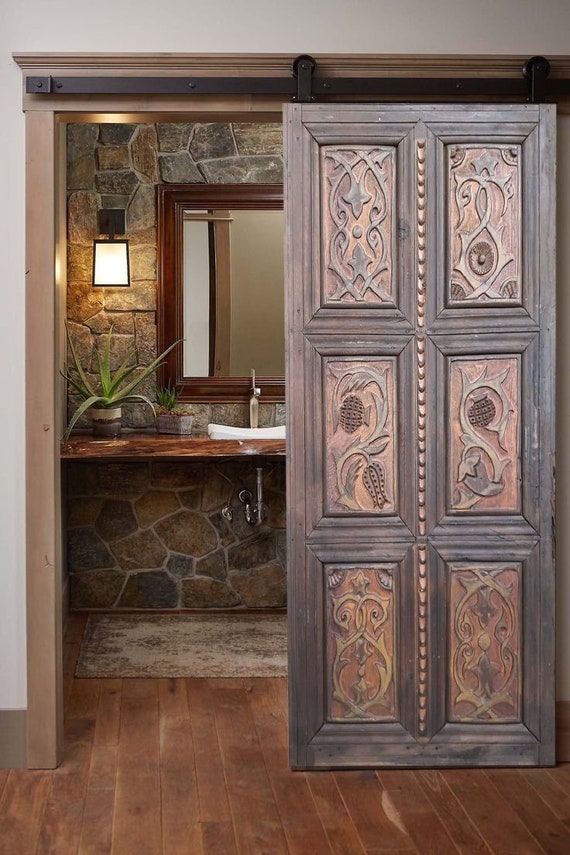This photograph captures the entrance to a bathroom, dominated by an ornate, six-panel wooden sliding door, suspended on rollers at the top. The door is intricately carved with floral patterns, featuring tree branches, pine cones, and leaves, combining a reddish-brown background with golden-colored wood for the designs. The door is roughly halfway open, revealing a rustic yet elegant bathroom interior. Behind the door, the bathroom showcases a robust sink counter made from a thick, dark-stained piece of wood, contrasted against a wall of large, earthy-toned stone bricks. A mirror hangs above the sink, complemented by a rectangular wall lamp. Adding a touch of nature, an aloe plant in an earthy-toned pot sits on the left side of the sink counter, enhancing the bathroom's natural, rugged aesthetic. A rug is placed on the wooden floor in front of the sink, completing the inviting and finely detailed ambiance of the space.